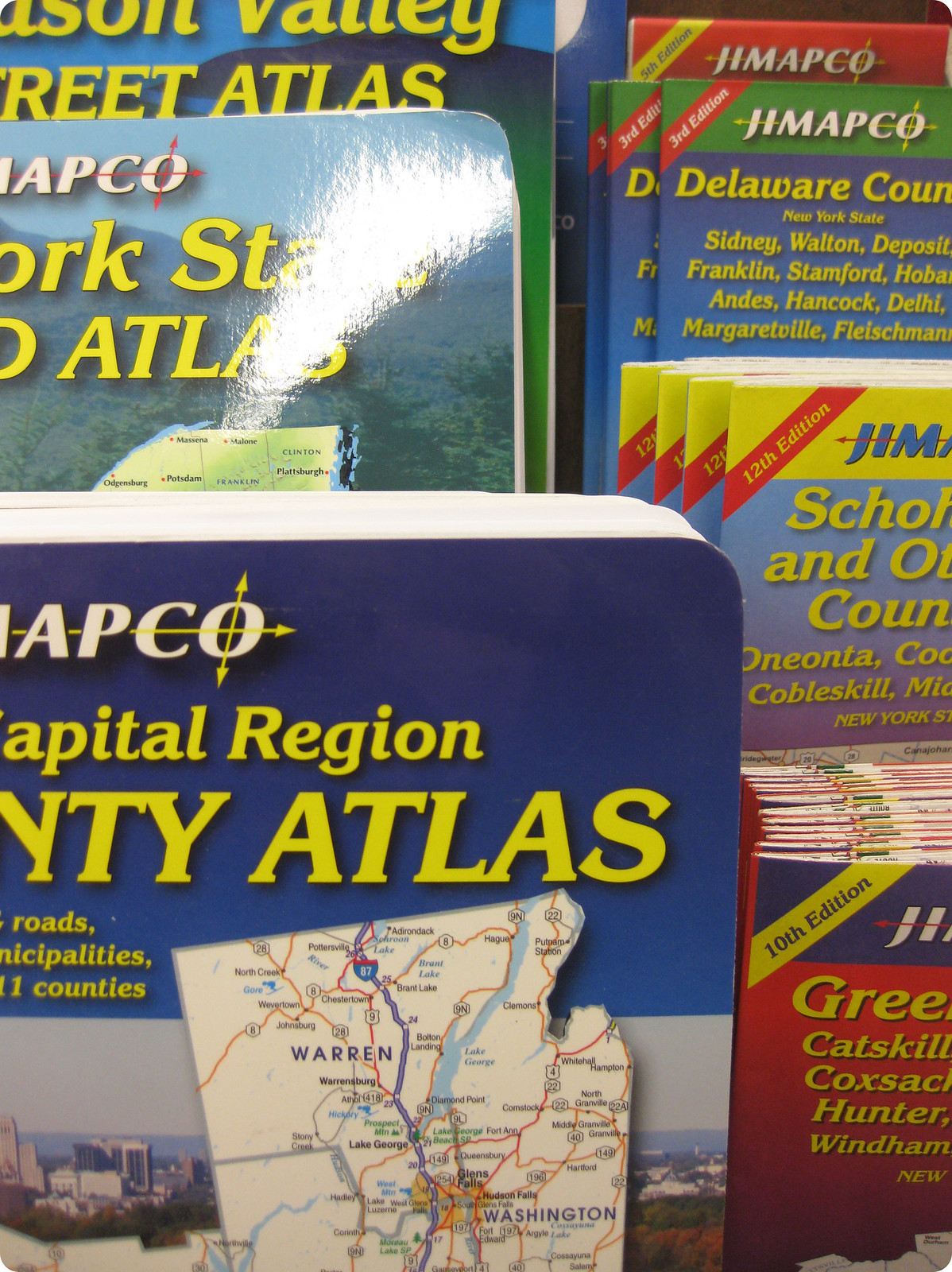This photograph showcases a detailed display case typically found in a travel-related building, perhaps a visitor center or a hotel lobby. The image zooms in closely on the display, revealing two distinct columns filled with various pamphlets and atlases. On the left side, prominently featured is a large atlas titled "Capital Region County Atlas" displayed above a visible map. Below it, pamphlets provide detailed information about Delaware County in New York State, listing specific towns such as Sidney, Walton, Deposit, Franklin, Stamford, Andes, Hancock, Delhi, Fleischmanns, and Margaretville.

To the right of these items, the display continues with more pamphlets, although the exact titles of some are partially obscured. Among them, a visible pamphlet references regions like the Catskills, specifically mentioning towns such as Coxsackie, Hunter, and Windham. The items on the right-hand side appear thinner, likely containing less detailed information than the larger atlas on the left.

The pamphlets and atlases overlap slightly within the display, creating a layered effect, indicative of a well-stocked resource area aimed at providing geographical and travel-related information for visitors interested in the Mid-Atlantic and New England regions. The detailed design includes blue and yellow lettering prominently featured on several materials, with one particularly notable pamphlet at the bottom right being blue and red with distinct yellow letters. This fraction of the display case clearly intends to guide travelers through the geographical intricacies of areas within the Capital Region and beyond.